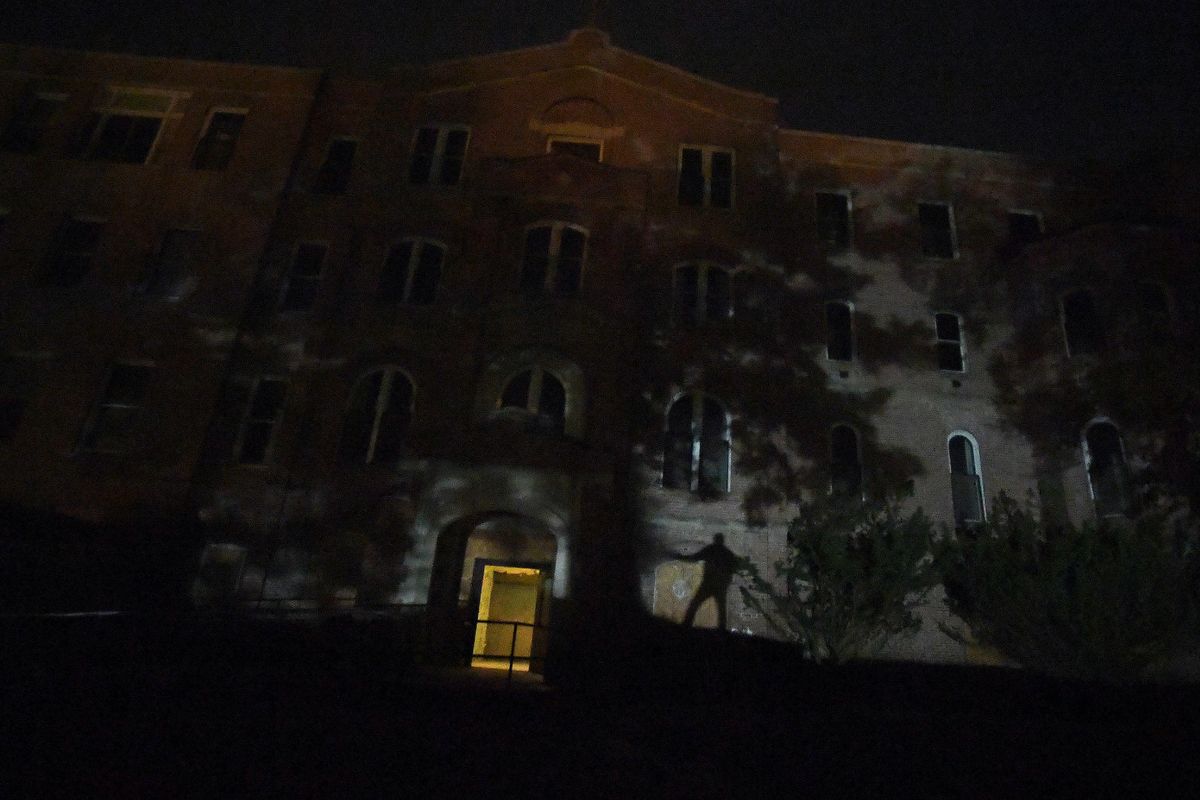In this haunting night-time scene, a large, three-story building, possibly a dormitory, school, or old institution, looms ominously against a black sky. Crafted from brick or stone and overgrown with ivy, the structure is cloaked in deep shadows, its many windows adding to its eerie presence. The building's entryway, set within a prominent arch, stands out with an unsettling golden glow illuminating the yellow door and casting dark, sinister shadows. To the right of the door, the chilling shadow of a man appears against the brick wall, adding to the horror movie-like atmosphere. Dim outlines of nearby trees and shrubs are visible, their shadows contributing to the sense of dread permeating the scene.